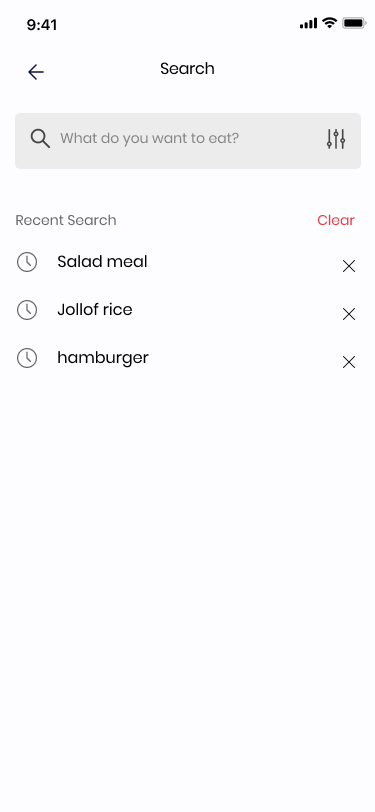This image depicts a screenshot of a mobile app interface. At the top of the screen, the time is displayed as "9:41," while the right side features fully filled standard status icons for Wi-Fi, cellular data, and battery life. Directly below this status bar, there is a thin black "back" arrow on the left side and the word "Search" centered in black text against an antique white background.

Below this header, there is a search bar with a gray undertone. It includes a magnifying glass icon and the placeholder text "What do you want to eat?" Within the search bar on the right side, there is a filter icon.

Further down, the screen is divided into two sections: the left side reads "Recent Searches" in black text, while the right side shows "Clear" in red text. Underneath these headers, the recent search results are listed: "Salad meal," "Jollof rice," and "Hamburger." Each search result is aligned to the left with a clock icon set to 4 o'clock. To the right of each result, there is an "X" icon, allowing the user to clear individual search history items.

The rest of the screen beneath these elements is blank, maintaining the antique white background, providing a clean and minimalistic user interface.